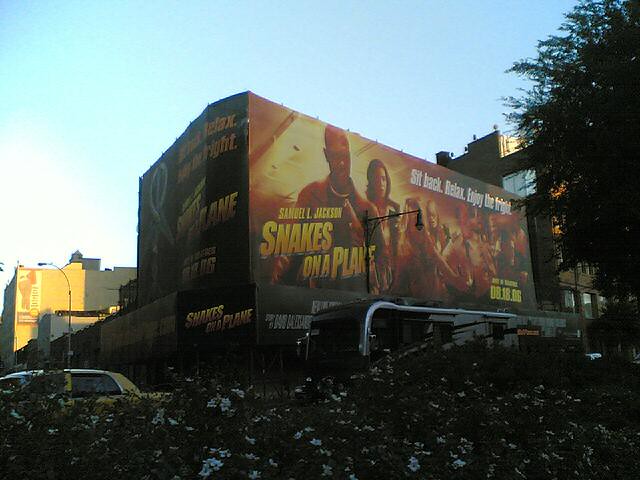This image features a billboard prominently displaying the movie "Snakes on a Plane." The billboard boasts bold yellow text, proclaiming the title alongside the name Samuel J. Jackson. The advertisement is somewhat blurry, making it challenging to discern finer details. At the center, there is an image of Samuel L. Jackson, identifiable by his bald head, glasses, and a choker-like necklace, coupled with what appears to be a red shirt. To his right, a group including a man and a woman can be seen, though their features are less distinct due to the blur.

The tagline "Sit back, relax, enjoy the fright" is written in white text. Beneath this, additional yellow text displays a date, "08-18-06," likely indicating the movie's release date. There is more text on the left side of the billboard, but it is unreadable.

Surrounding the billboard are urban elements: buildings are visible in the background, with more structures to the left. A tree stands on the far right, accompanied by an assortment of plants and flowers at the base of the billboard. A silver bus is in the background, its windows faintly visible, and to the left of the bus, a car is also present. The scene is set against a backdrop of a clear, blue sky.